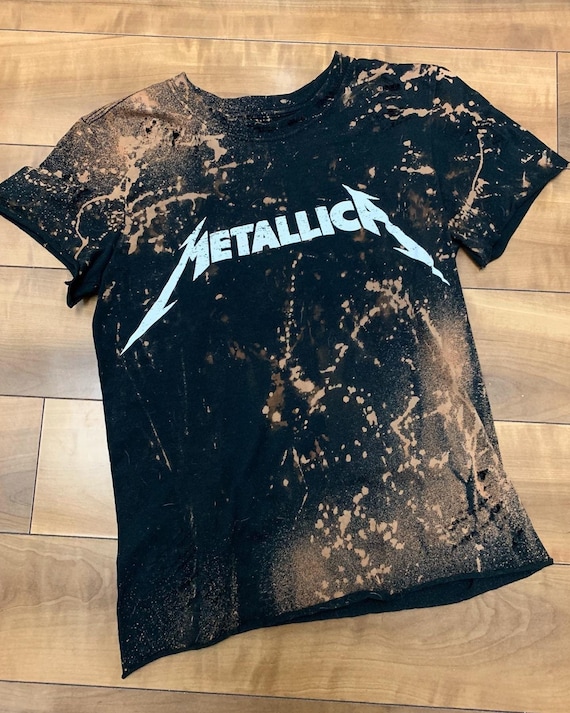The image showcases a black Metallica t-shirt laid flat against a medium brown wooden floor. The shirt features the iconic Metallica logo prominently across the chest in white. Adding a unique twist to its design, the shirt has been artistically splattered with bleach, resulting in an array of brown tan dots and mist-like patterns. Notable areas with heavier misted bleach marks include the bottom right corner and the upper left shoulder, suggesting the use of a spray bottle. The shirt’s placement and distinctive bleach patterns lend it a striking, edgy appearance that could appeal to both men and women.